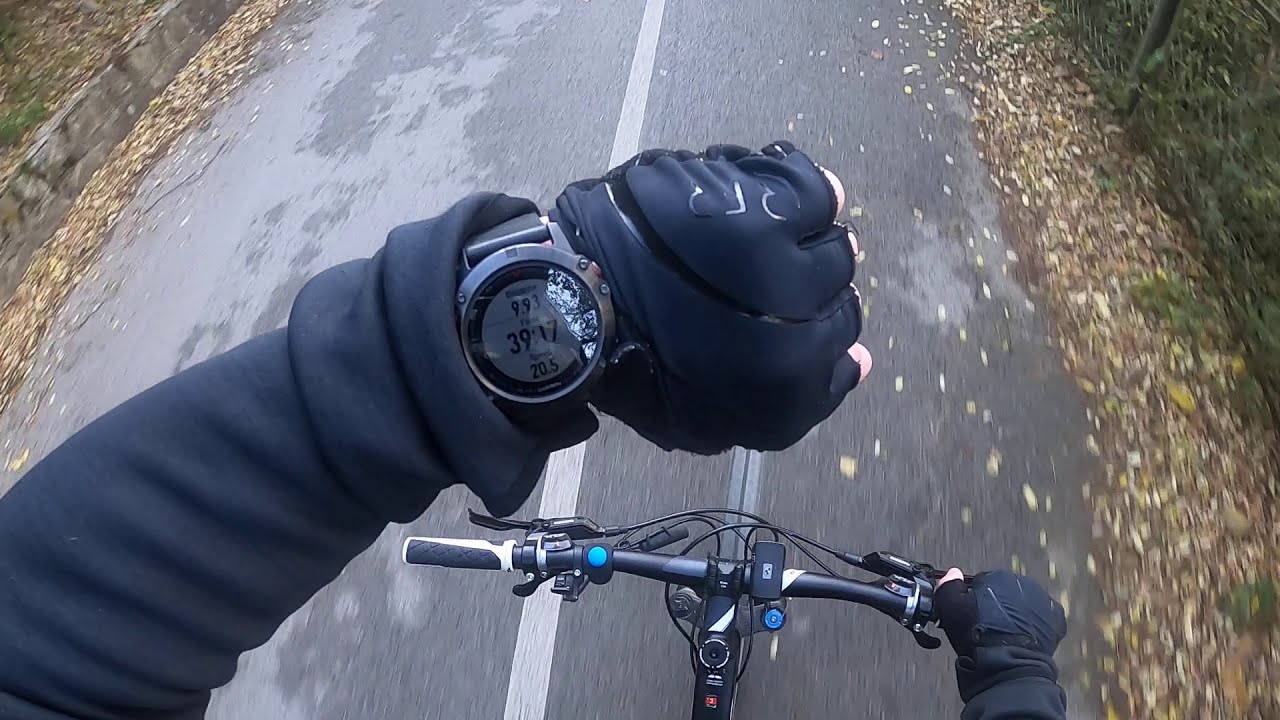This horizontal, rectangular image appears to be taken from the perspective of a GoPro mounted on the helmet of a cyclist. The photograph captures the cyclist riding forward on a paved bike path characterized by a centered white line. The cyclist’s right hand is gripping the black handlebar, which features some blue buttons, and the left hand is raised, checking a round, digital-display watch. The individual is dressed in a long-sleeved, dark-colored jacket or possibly a leather sweater, with the sleeve pulled back to reveal the watch. Dark blue, fingerless gloves cover their hands. 

The path, wide enough for bicycles but not cars, is bordered by an array of fallen leaves in shades of yellow and brown, indicating it is likely autumn or a chilly time of year. The environment includes trees and brush lining the sides, with grass visible amongst them. The colors in the image primarily comprise dark blue, white, gray (from the asphalt), along with the natural hues of brown and green. No other people or animals are visible in the scene.